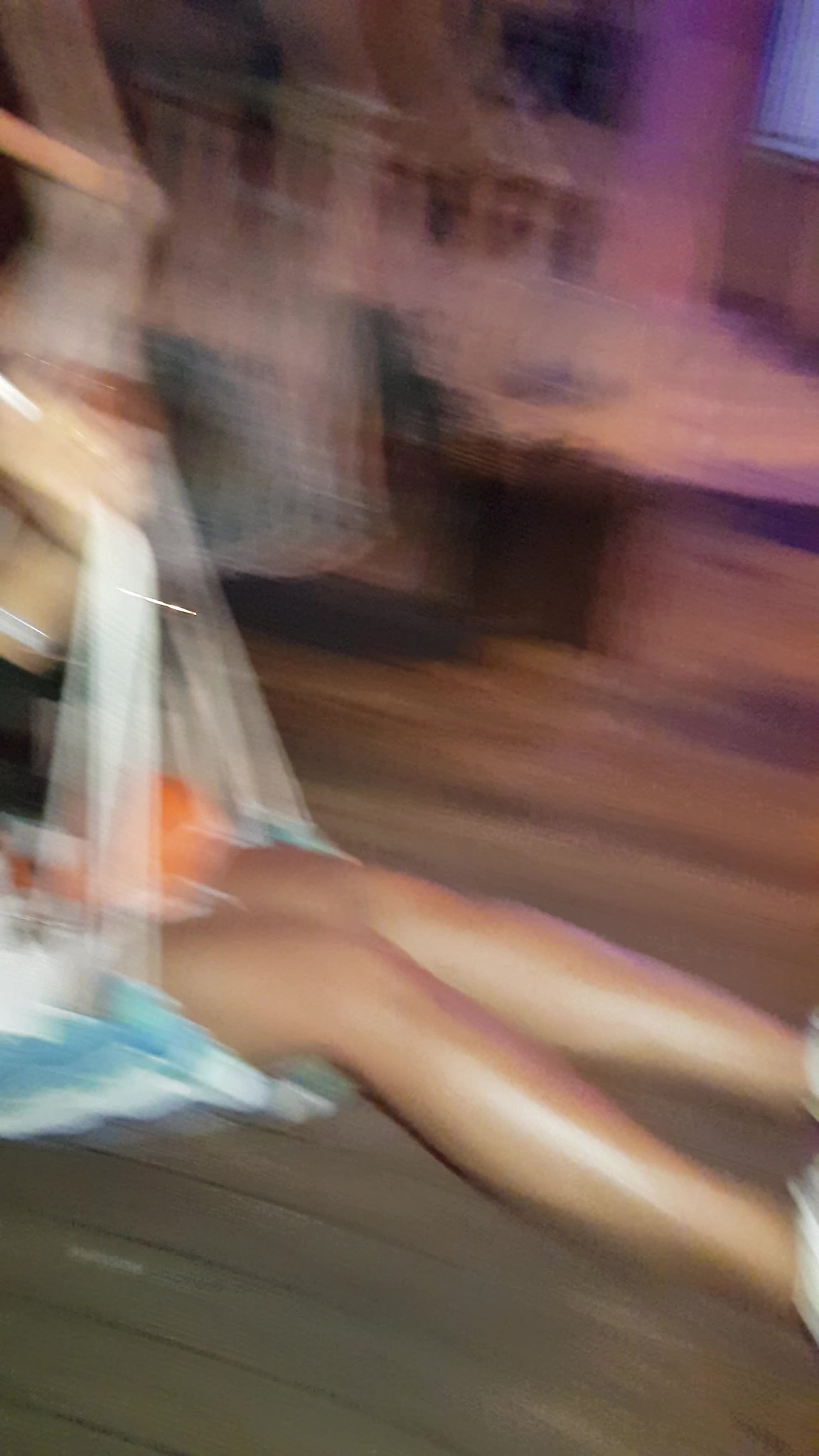This color photograph, although extremely blurry and difficult to discern, appears to have been taken outdoors, possibly during motion or in low light conditions. The dominant colors in the image are purples and browns, contributing to its unclear quality. In the lower half of the picture, there seems to be a wooden porch with brown boards. The most distinguishable feature is a pair of legs in the foreground, clad in white tennis shoes and white and orange shorts, indicative of a medium complexion person. These legs seem to be seated in a swing, with a white and light blue patterned basket made of some fabric. The swing, featuring white strings, extends to the top left corner of the image. The background shows additional blurry figures, possibly people on similar swings, suggesting this could be a scene at an amusement park or carnival.